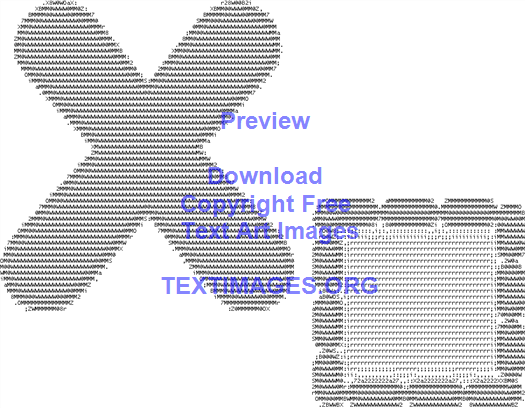The image appears to be a promotional or splash screen for ordering art images online and features a clean white background. Prominently displayed in the upper left corner is a needlepoint-textured black and white "X," creating a large gray X effect. Positioned in the lower right corner is a square bordered by a darker frame made of cylindrical shapes, with a lighter gray and white needlepoint interior. Over these needlepoint graphics, there is blue sans serif text that reads in sequence: "Preview," "Download," "Copyright Free," and "Text Art Images." Below these lines, in larger blue capitalized text, the website "TextImages.org" is displayed. The overall aesthetic is minimalistic and pixelated, combining intricate needlepoint textures with modern typography.